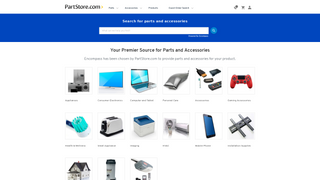A screenshot of the homepage of a website, likely named "partstore.com," offering a variety of electronics and accessories. The page features a search bar at the top, followed by the slogan "Your premier source for parts and accessories" in black print. Below the slogan are three rows of product thumbnails. The first row includes six clickable items, as does the second row, while the third row has only three items displayed due to being partially cut off in the image. Visible products include gaming systems, TV monitors, USB charging devices, Xbox controllers, electric toothbrushes, toasters, cellphones, and TV mounting equipment. The titles under the third-row items are not visible, suggesting the image is cropped. The overall layout indicates a diverse range of household and electronic products.